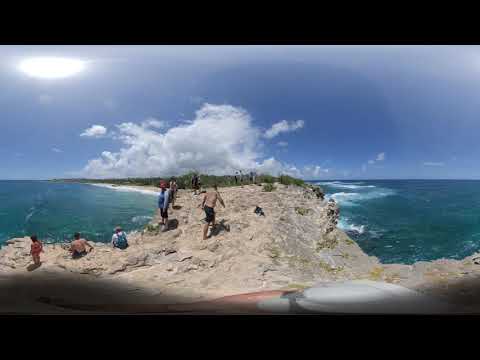The image captures a vibrant beach scene on an island in Hawaii, under a brilliant blue sky adorned with a few scattered white clouds and the bright sun shining from the top left. In the foreground, beige rocks create a natural platform that visitors are using to jump into the crystalline blue water. Three people are positioned at the edge of the rocky area: one is standing while the other two are seated. One of the seated figures is a girl wearing bibs and a white t-shirt, while the others are shirtless. A man in black shorts can be seen running, seemingly ready to leap into the ocean. To the left, several people sit on the rocks, overlooking the serene scene, while others wait their turn to jump. The center of the image features lush greenery leading to a pristine, white sandy beach. To the right, the open ocean displays gentle waves washing up against the rocks, with a few individuals enjoying the water. Overall, the picture evokes a relaxed, vacation atmosphere where people leisurely enjoy the natural beauty of Hawaii.